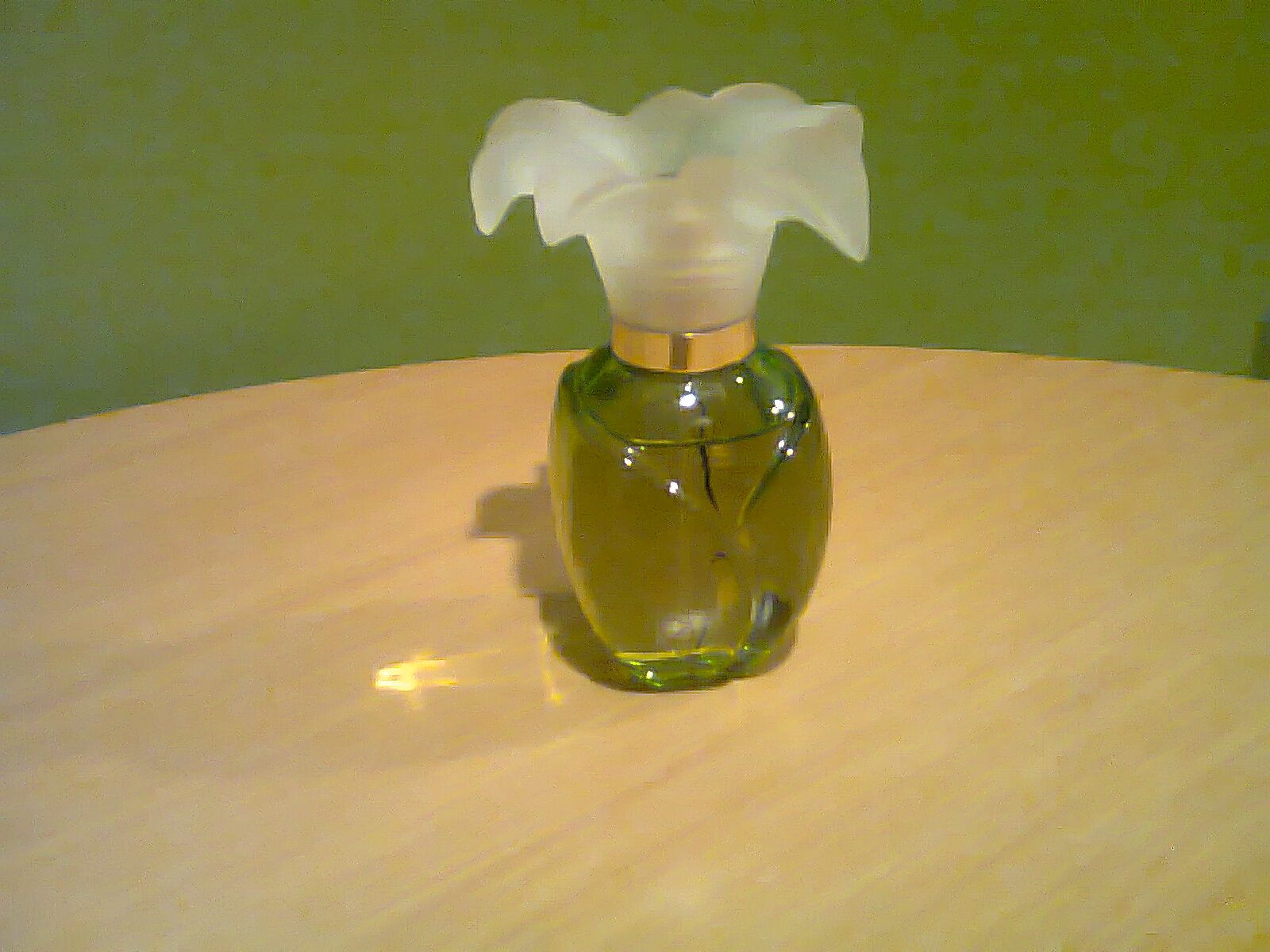This indoor colored photograph features a scene with a bright green background dominating the upper portion. Centrally positioned on a round, light brown, almost tan wooden table, there is a distinctive glass bottle. The bottle, short and bubbly, tapers at the bottom into a round, smooth shape and appears either green-tinted or filled with green liquid. As light reflects through the glass, it creates a gleaming effect on the table's surface. The bottle is adorned with a gold rim around the neck and topped with an intricately designed lid resembling an open white flower. This flower-shaped lid appears to be made from frosted, sanded glass or plastic, adding an element of delicate charm to the overall composition. The bottle, measuring about two to three inches tall, has an ambiguous purpose, possibly serving as a perfume container or an air freshener.